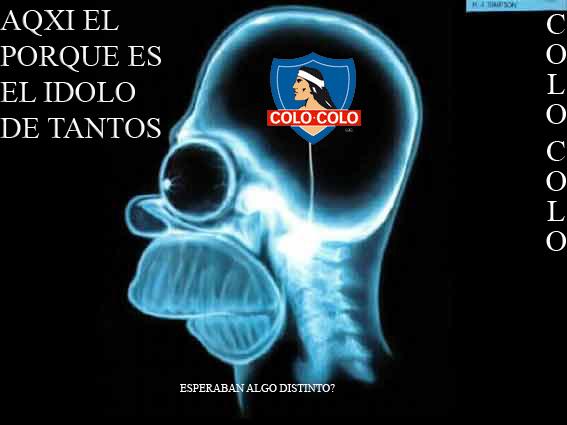The image appears to be an x-ray scan of Homer's head, showcasing his teeth, eyeballs, nose, and neck vertebrae. Notably, within the center of his skull, where his brain should be, there is an intricately designed shield. This shield features a depiction of a Native American male with long hair and a headband, etched in white against a blue background. Below this image, there is a red vertical bar labeled "Colo Colo" in white letters. The top left corner of the image contains unreadable Spanish text, beginning with "AQXI EL, PORQUE ES, EL IDEIDOLO, DE TANTOS," and additional white text on a black background at the bottom reads "ESPERABAN ALGO DISTINTO." Both the large eye sockets and exaggerated jawline further emphasize the resemblance to Homer Simpson.